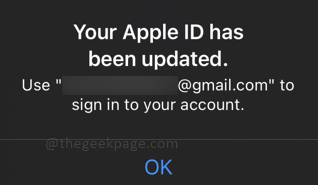A black rectangular notification, measuring approximately 5 inches in width and 4 inches in height, contains a message in white text. The message reads: "Your Apple ID has been updated." The "I" and "D" in "ID" are capitalized for emphasis. Below this, the text instructs, "Use '[redacted]@gmail.com' to sign in to your account." The placeholder "[redacted]" is used to obscure sensitive information, shown as a blacked-out rectangle. Centered approximately 2 inches below this text, the word "OK" appears in blue, indicating a button to acknowledge and dismiss the notification.